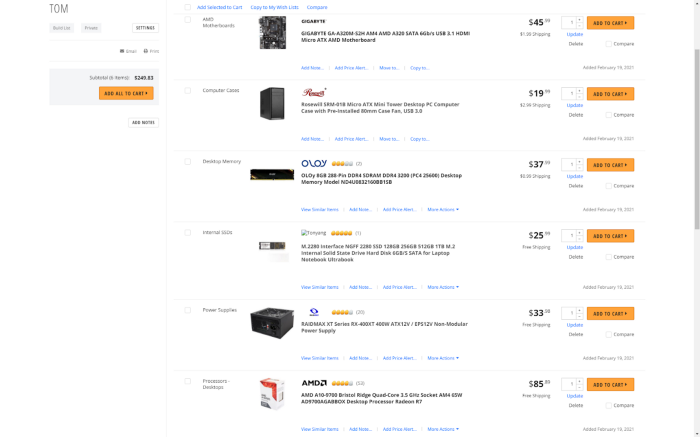A screenshot from an unidentified PC parts website is displayed. In the upper left corner, the word "Tom" is prominently featured. Below this, there are several grey-on-grey buttons with illegible text, except for one white-on-black button labeled "Settings." The browser also shows Gmail and another application, as well as a shopping cart subtotaling $249.83.

On the right-hand side, a selection of PC components is listed. These include a black Gigabit motherboard, a black PC case, a stick of RAM, an M.2 SSD, a black power supply, and a white-and-red boxed AMD CPU. The listed prices for the items are $49.99, $19.99, $37.99, $25.99, $39.95, and $85 respectively. The commentator notes that the computer may not perform well due to the cheap power supply.

The interface includes black buttons with orange text labeled "Add all to cart" and individual "Add to cart" options. On the upper right, there's a vertical scrollbar about a quarter of the way down, depicted in a darker grey. The overall tone suggests a critical view of the selected components.